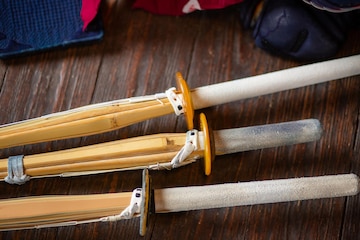This image depicts three objects resembling faux Japanese swords, displayed horizontally on a textured mahogany-style wooden table. The objects feature intricate wooden handles on their left sides, comprised of light-colored brown wooden strips bound together with cords and possibly duct tape. Each handle transitions into a round guard, evoking traditional samurai sword design. Beyond the guards, the 'blades' are made from white, spongy Styrofoam, with two being longer and one shorter in the middle. At the right end of the objects, a white Styrofoam segment protrudes, reminiscent of a candle. Surrounding the swords on the table are indiscernible objects, including black, red, and blue items, one of which seems to be a red shoelace or piece of cloth. The overall scene presents an intricate array of textures and colors, enhancing the unique visual appeal of the display.